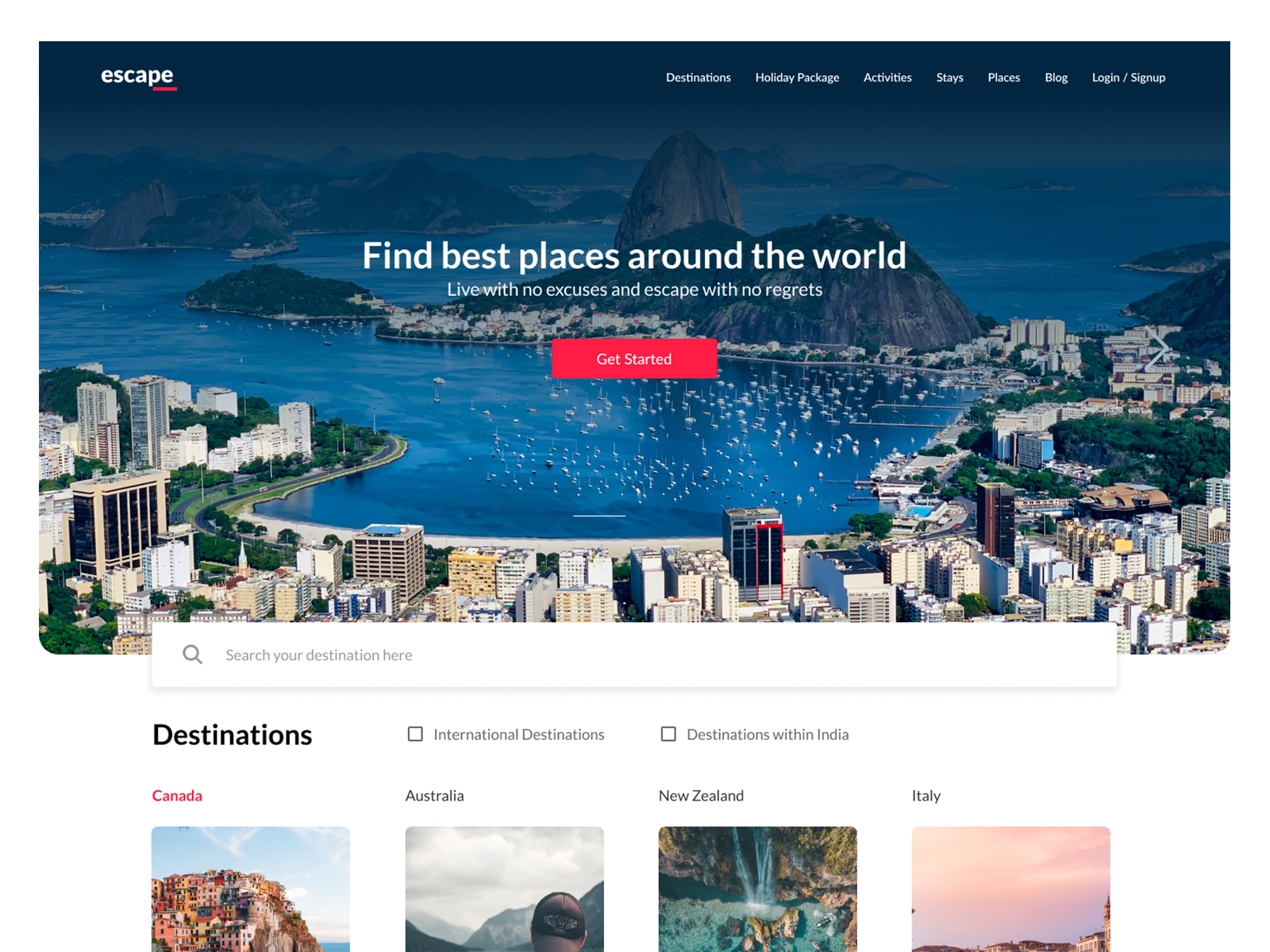**Caption: Exploring the Perfect Escape**

The screenshot features a vibrant blue backdrop, resembling an aerial view over the tops of buildings, transitioning into water with a small mountain in the center and larger mountains in the distance. Centrally positioned in bold white text, it reads, "Find best places around the world." Below, in smaller white font, it states, "Live with no excuses and escape with no regrets." A horizontal red rectangle with white text inside urges viewers to "Get Started."

In the upper left corner, the word "Escape" is highlighted with the letters "PE" underlined. Slightly right of center are clickable options in white: "Destination," "Holiday Package," "Activities," "Stays," "Places," "Blog," and "Login/Sign Up."

At the bottom, a pop-up window presents a search bar outlined in gray with a magnifying glass icon on the left, prompting, "Search your destination here" in small gray text. Below that, bold black text labeled "Destinations" features two checkboxes: "International Destinations" and "Destinations within India." Four partially visible images at the bottom are labeled "Canada" (in red), "Australia," "New Zealand," and "Italy."